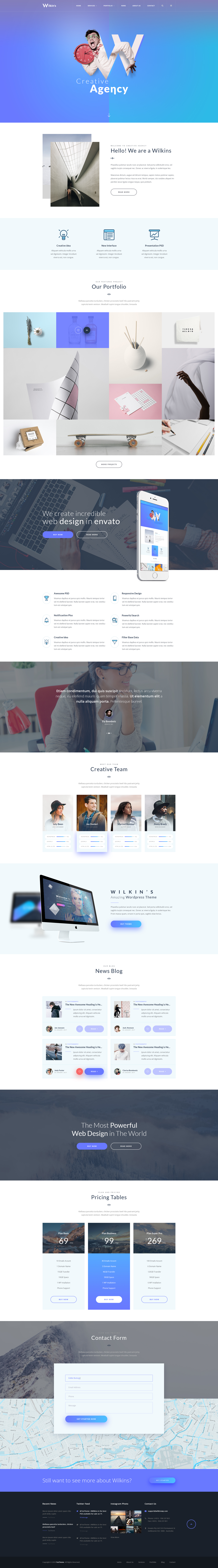In the image, the background is a gradient of light to dark blue, creating a visually appealing backdrop. There are two main images featured prominently. One image shows a face and a portion of a "V", likely representing a person's portrait or a logo. 

At the top of the image, the text "Hello, we are Wilkins" is displayed in a bold white font. Below this header, there are three distinct icons in a horizontal row, each designed to draw attention. The color scheme across the images and elements includes shades of blue, dark blue, white, and pink, adding vibrancy to the overall design.

In the lower section, a skateboard is visible, adjacent to a red object that isn't clearly identifiable. Near these items, the word "design" is prominently displayed, perhaps suggesting the type of work or theme being illustrated. A smartphone appears next to these elements, placed in front of a gray background that transitions into a visual of a laptop displaying text and an icon. The edges of the image seem to fade into gray, providing a subtle border to the composition.

Highlighted in a blue oval are the words "The most powerful word design in the world." Below this, there appears to be sections dedicated to pricing tables and a contact form. At the bottom of the image, a black bar includes some additional text, while a blue bar above this features more content, creating structured and organized segments within the design.